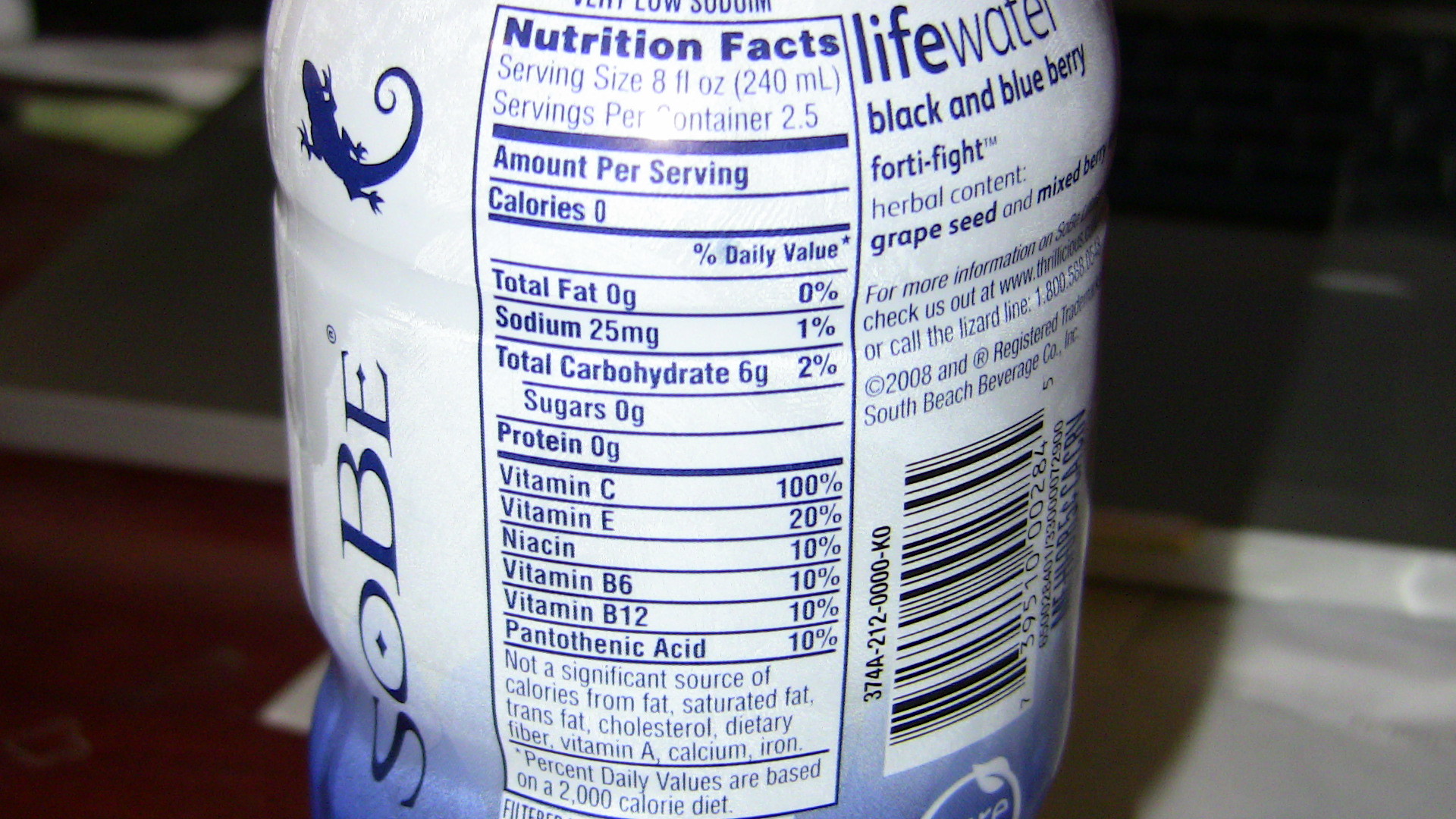The image is a close-up photograph of a nutritional label on a Sobe brand beverage bottle. The bottle, which has an ombre design transitioning from blue at the bottom to white at the top, is perched on an indistinct surface in the background. Dominating the label is the Sobe brand name in blue text, accompanied by a dark blue lizard with a distinctive curly tail in the top left corner. To the right, the label prominently features the product name "Life Water," with the specific flavor indicated as "Black and Blueberry." Additionally, the label highlights that the drink is "Fortified" and contains "Herbal Content," "Grapeseed," and "Mixed Berry," though the latter word is partially cut off.

The nutritional facts listed in blue text on the white background provide detailed information, including zero calories, zero fat, 25 milligrams of sodium, six grams of total carbohydrates, zero grams of sugars, and zero grams of protein. Vitamins are prominently featured, including 100% of the daily value for Vitamin C, 20% for Vitamin E, 10% for niacin, 10% for Vitamin B6, 10% for Vitamin B12, and 10% for pantothenic acid. A vertical barcode is situated on the bottom right of the bottle.